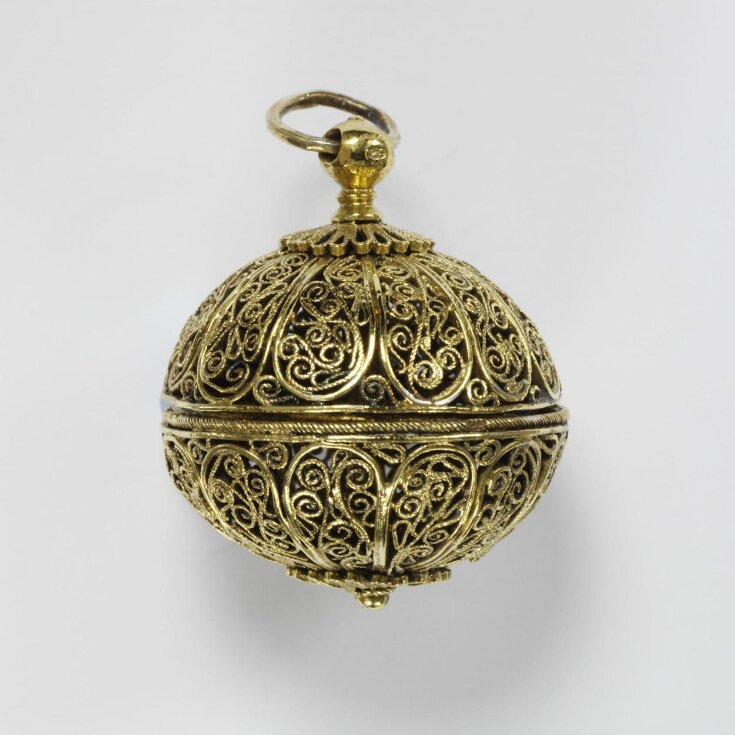The image depicts a vintage, intricately designed ornament set against a solid gray background. The ornament features a circular, gold and brown design, exuding an antique feel reminiscent of craftsmanship from the 1960s. Central to the decoration is a detailed pattern of swirling lines, both large and small, forming a harmonious and repeated motif across its surface. The piece is divided into two symmetrical halves, with horizontal lines connecting the top and bottom semi-circles. At the ornament's apex is a small round ball with a hole through which a circular ring is attached, allowing the piece to be hung or worn. The ornament, possibly made from gold and brass, appears both valuable and versatile, resembling something that could serve as a fine pendant, a decorative knob, or a cherished Christmas decoration.